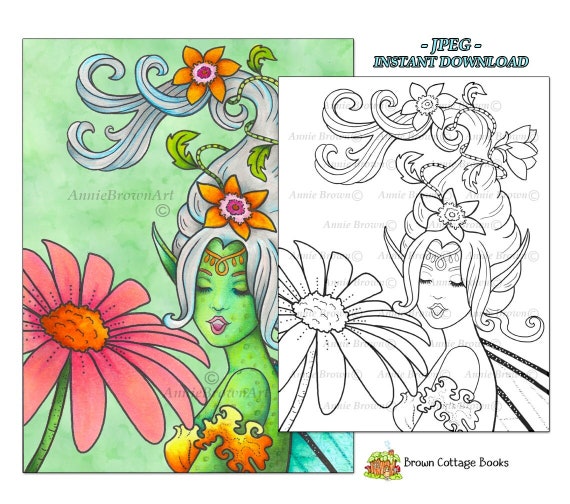In this up-close coloring book-style photograph, two images are displayed side by side: one colored in and the other an identical black-and-white version ready for coloring. The background of the colored image is a hazy green. Centered within both images is a female sprite or elfish character with green skin, standing sideways with her left shoulder facing the viewer, her head turned towards the front. Her long, grayish-blue hair extends upward and curls slightly, adorned with twirling vines and orange and pink flowers. Notably, a vibrant orange flower blooms above her brow, and she wears a yellow headband and a crown-like crest. Her eyes are closed, her mouth open, and she dons pink lipstick. A red, fiery plant-like blouse covers her upper body, accented by a band around her upper arm resembling flames. To the left of her, there is a large daisy with hot pink petals, an orange center, and a dark green stem. The black-and-white version sits slightly overlaid on the colored one, with a watermark reading "Annie Brown Art" to prevent unauthorized use. Additionally, a "JPEG Instant Download" caption appears at the top right, and at the bottom, an emblem of a cottage with a green roof accompanies the text “Brown Cottage Books.”